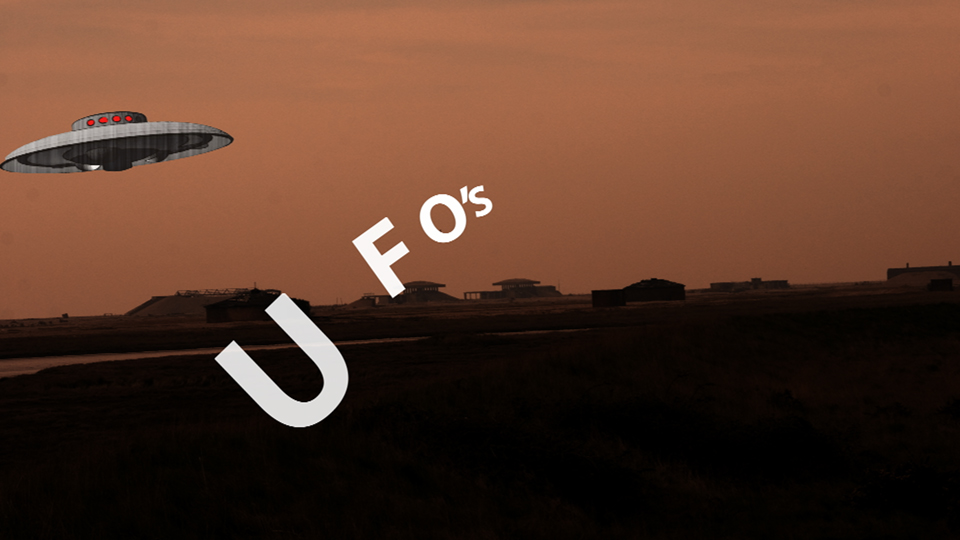In the image, a scene is presented with a striking, Mars-like reddish sky occupying the top half, juxtaposed against a dark, night-time landscape that covers the bottom half. The landscape includes silhouettes of buildings or possibly an airbase, and a field, creating a stark visual divide. A prominent feature is the digitally placed, classic gray flying saucer with a black base and four glowing red dots, positioned in the top left corner, hinting at a UFO. The sky appears almost as if it has a sepia or light coffee tint, further enhancing the otherworldly atmosphere. Central to the composition, and slightly left of center, the white text "UFO's" is angled upward to the right, with noticeable spacing between the letters, particularly wide between the "U" and "F" and more compact toward the end. This text stands out sharply against the murky background, adding to the mysterious aura of the scene.